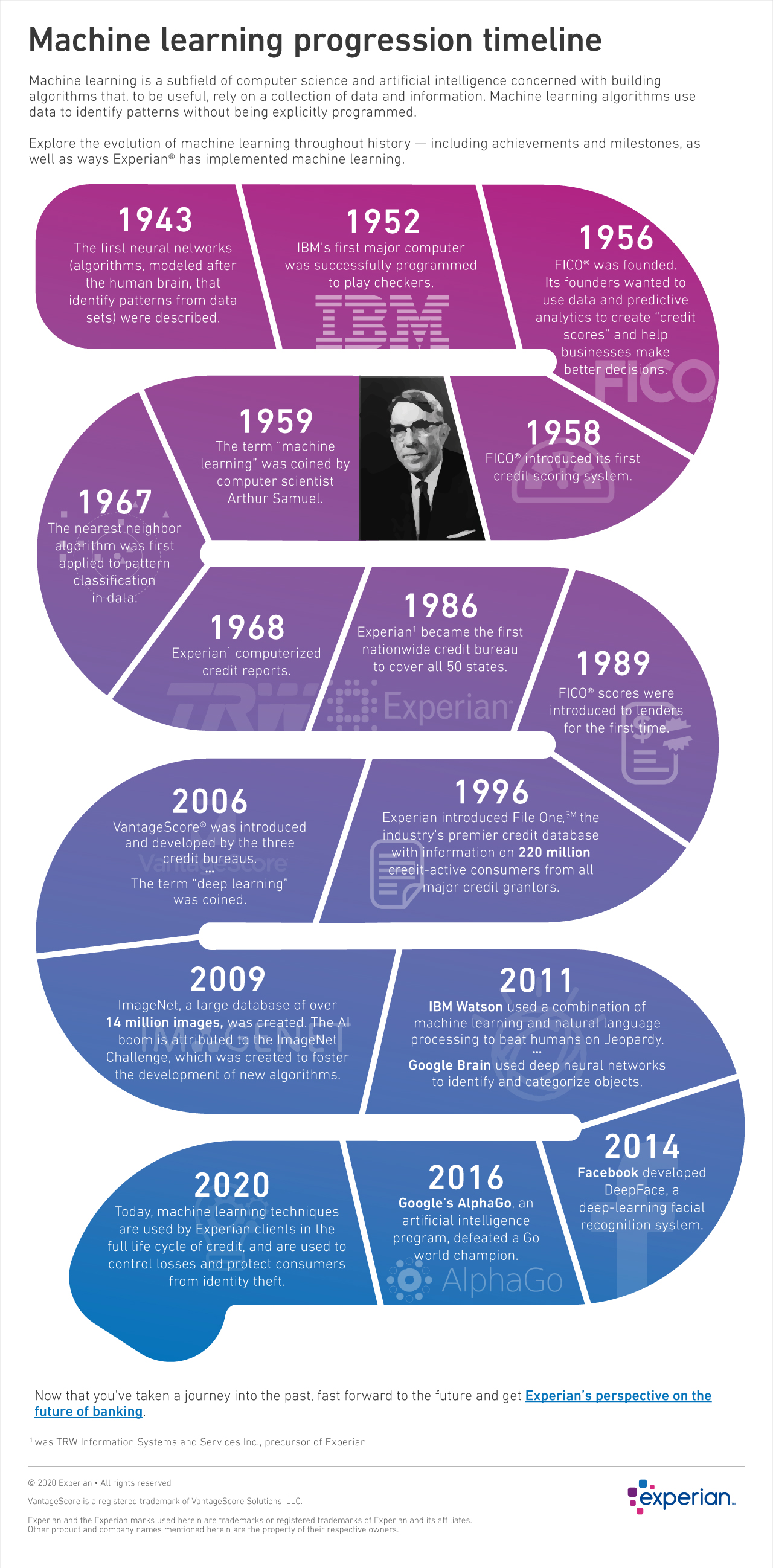The image displays a colorful, detailed timeline titled "Machine Learning Progression Timeline," showcasing the evolution of machine learning from 1943 to 2020. This timeline, designed in a serpentine, S-like shape and gradient color that transitions from bright purple at the top to blue at the bottom, highlights key milestones in the development of machine learning. The diagram includes important dates and events, such as 1952 where IBM made contributions, and 1959 where the term "machine learning" was coined by computer scientist Arthur Samuel, whose photo is also featured. Along the way, it annotates various significant advancements and achievements within the field. The bottom right corner features the Experian logo, indicating their involvement and implementation of machine learning techniques, particularly in credit lifecycle management and identity theft protection. While the text is dense with detailed information, it is somewhat difficult to read, and likely includes links to further resources at the bottom.